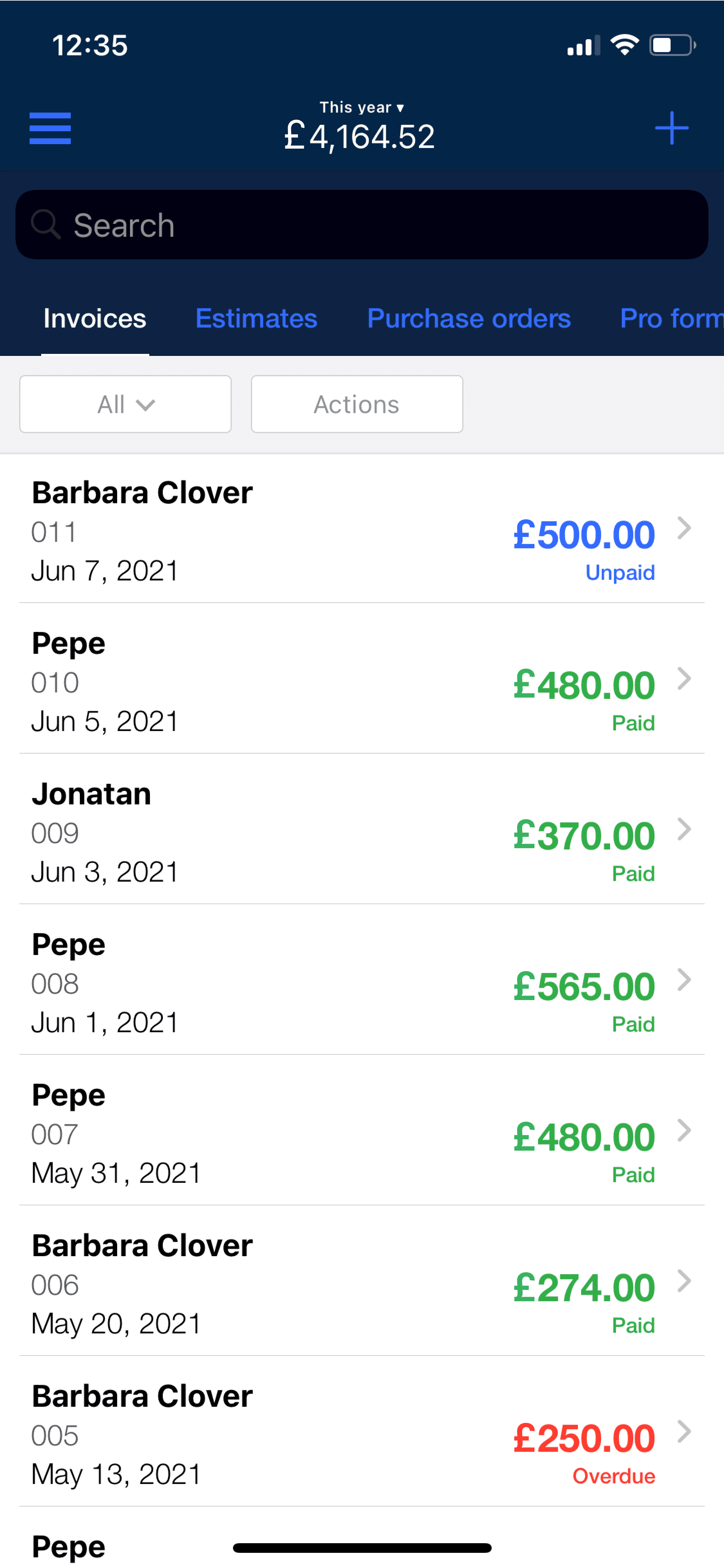The image is a detailed screenshot of a transaction management interface with the currency set in British Pounds. At the very top, it shows the account holder's current balance, which stands at £4,164. Directly below this, there is a prominent black search bar. Below the search bar are four distinct options labeled: Invoices, Estimates, Purchase Orders, and Pro-Forms.

The main section of the screenshot features a comprehensive list of individuals or organizations involved in financial transactions, with their respective names and status of payments displayed. Notable names include Pepe, Barba Clover, and John Jonathan. On the right side of each entry, the amounts are listed, color-coded for clarity: some are in green (indicating paid status), one is in blue, and another in red (possibly indicating different statuses like unpaid or overdue). Specifically, one entry is marked in red as 'overdue,' while another is at the very top labeled 'unpaid.'